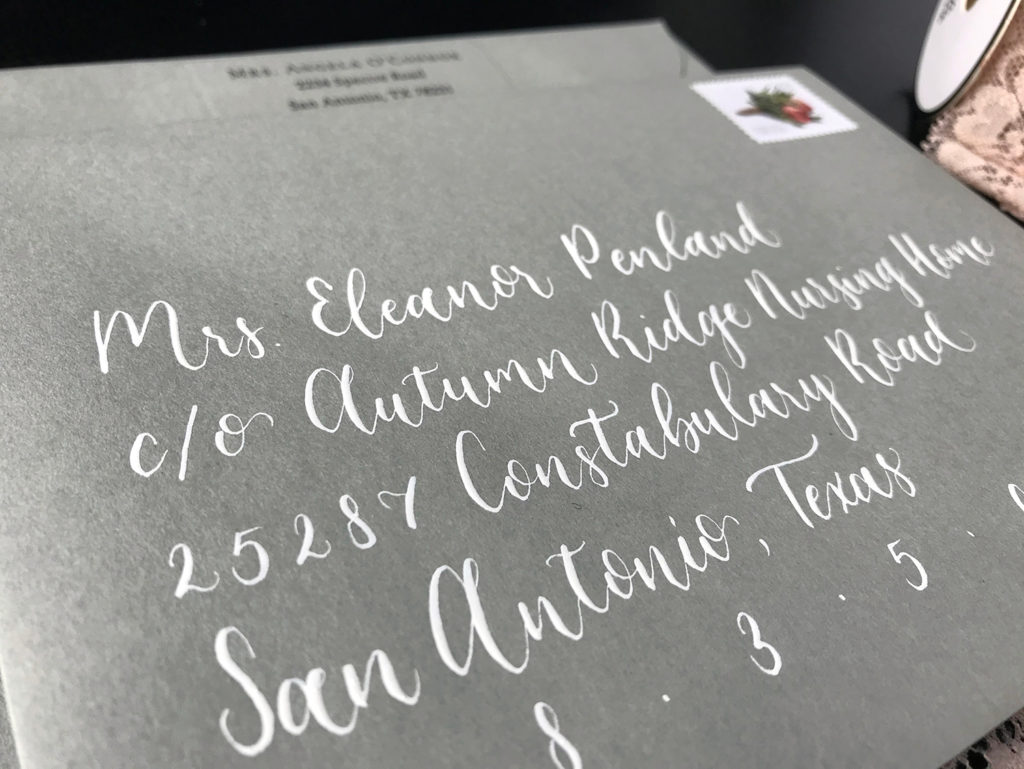The image depicts a dark-colored envelope, possibly black or gray, with intricate white cursive text printed on it. The address reads: "Mrs. Eleanor Penland, C/O Autumn Ridge Nursing Home, 25287 Constabulary Road, San Antonio, Texas." The zip code starts with "835" but is partially obscured. In the top right corner, there is a white stamp featuring a blurred image that appears to be a flower or fruit with green leaves. Overlapping this envelope is another of similar color, visible at the top edge.